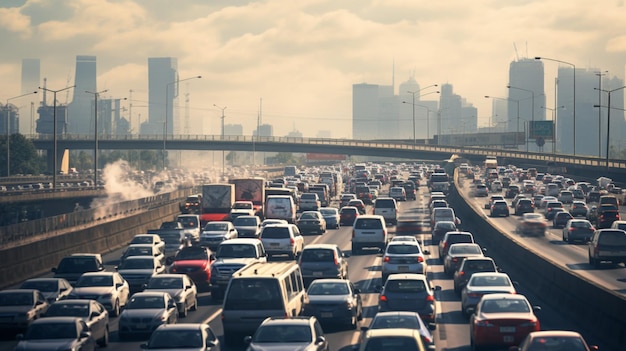This image captures a bustling urban highway, densely packed with vehicles, including cars, trucks, and vans predominantly in white, red, blue, and black. The highway, which stretches from the bottom of the image to about two-thirds up, is divided into multiple lanes heading away from the viewer. Two sets of lanes in the middle are moving in the same direction, while other lanes on the sides are directed differently. A bridge spans over the highway, although it's unclear if it accommodates pedestrians or traffic. On the left side, smoke or steam is emanating from an indistinguishable source off the highway. Further into the distance on the right, a green traffic sign is visible, though too small to discern its exact message. Numerous light posts line the highway and are visible in the background. The backdrop is dominated by hazy, fog-covered skyscrapers, adding to the congested and somewhat obscured urban skyline.